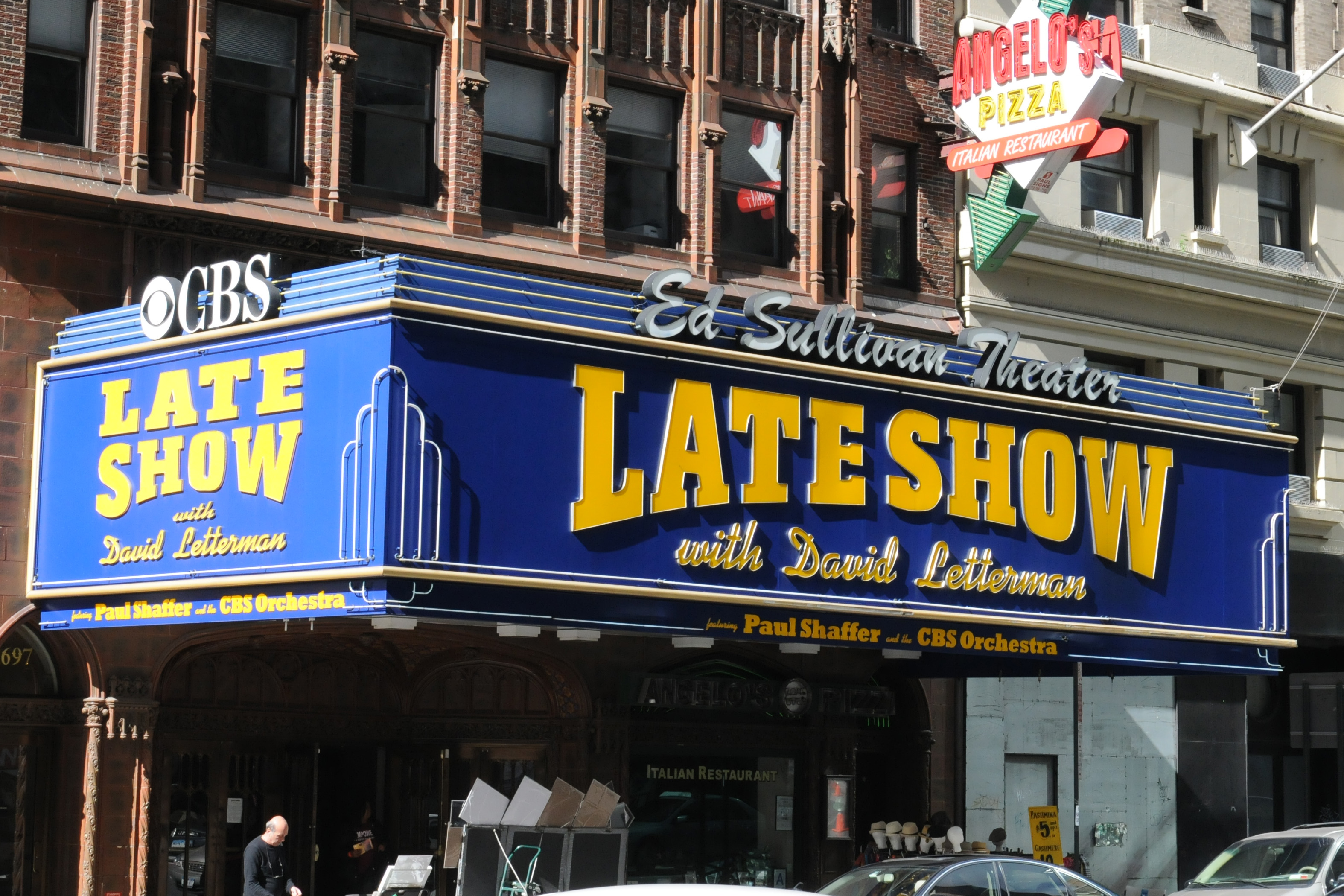This color photograph, captured in landscape orientation, vividly depicts the iconic entrance of the Ed Sullivan Theater. The marquee, a large blue rectangular canopy, dominates the scene with prominent gold lettering. At the front, the marquee reads "Late Show" in an athletic font, angled upwards, with "With David Letterman" beneath it in an elegant script font. Across the top, "Ed Sullivan Theater" is inscribed in a white brush font, standing out prominently.

On the left side of the marquee, the CBS logo and the word "CBS" appear in white, followed by "Late Show with David Letterman" in yellow letters on a blue background, accompanied by "With Paul Shaffer and the CBS Orchestra" in smaller gold letters. Above the marquee, a red brick building with numerous windows provides a contrasting backdrop, while a sign for Angelo's Pizza, featuring a white pizza box and a green arrow pointing down, juts out from the building. This sign is clearly visible alongside a neighboring white building.

Below the marquee, several shops are visible, and on one of the windows, the words "Italian restaurant" can be discerned. In the foreground, a few cars are parked at the curb, adding to the everyday city atmosphere. The photograph captures the bustling essence of this famous New York City location, blending architectural details and urban life.